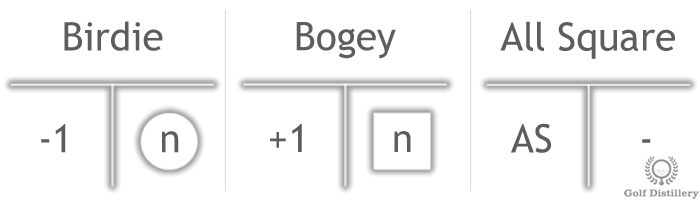The image consists of three vertically aligned sections on a white background, each divided by a T-shaped formation into two columns, with light gray text and details prominently displayed in black. 

The left section is labeled "Birdie" at the top, with a minus one (-1) on the left side of the T's post and an 'N' enclosed in a circle on the right side. 

The middle section is marked "Bogey," with a plus one (+1) on the left and an 'N' within a square on the right. The term "All Square" titles the right section, where an "A.S." appears to the left of the T and a simple horizontal dash lines up to the right.

At the bottom right corner of the image, there is a small logo reading "Golf Distillery," though it is somewhat difficult to read due to its size. This formation spans horizontally across the image, presenting a systematic golf scoring notation.